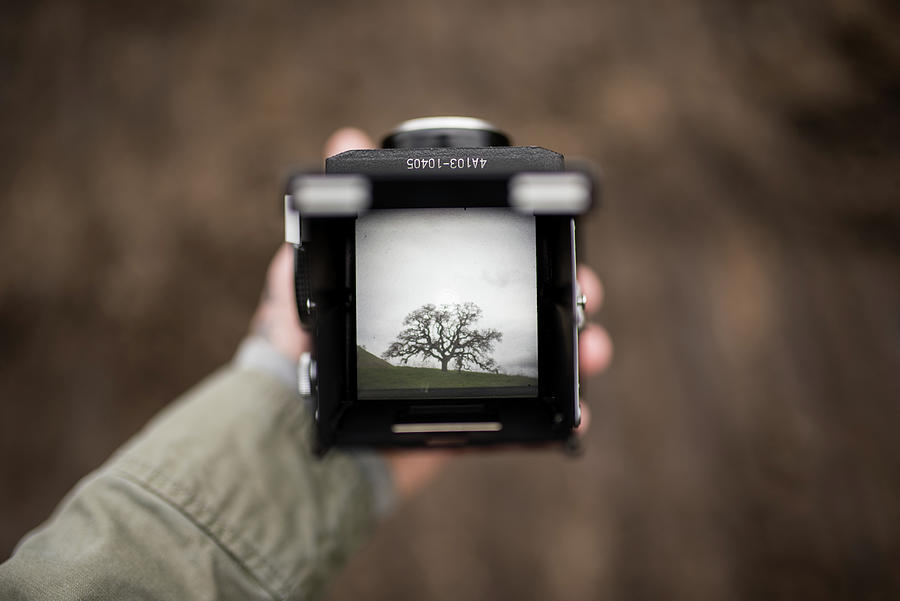In this outdoor image, a Caucasian hand with a beige skin tone, emerging from the bottom left of the frame, holds a black digital camera. The person's arm is clad in a gray, long-sleeved shirt. The camera's screen displays a picturesque scene: a large, leafless tree with numerous branches spreading outwards, rooted in a green grassy slope that inclines gently to the left. The backdrop features a gray, overcast sky. The background outside the camera's screen appears blurry, filled with indistinct shades of brown, black, white, and beige, indicating an outdoor setting. The picture is bright, suggesting daylight, and some digits – 4A103, 104, 05 – are seen on the camera.